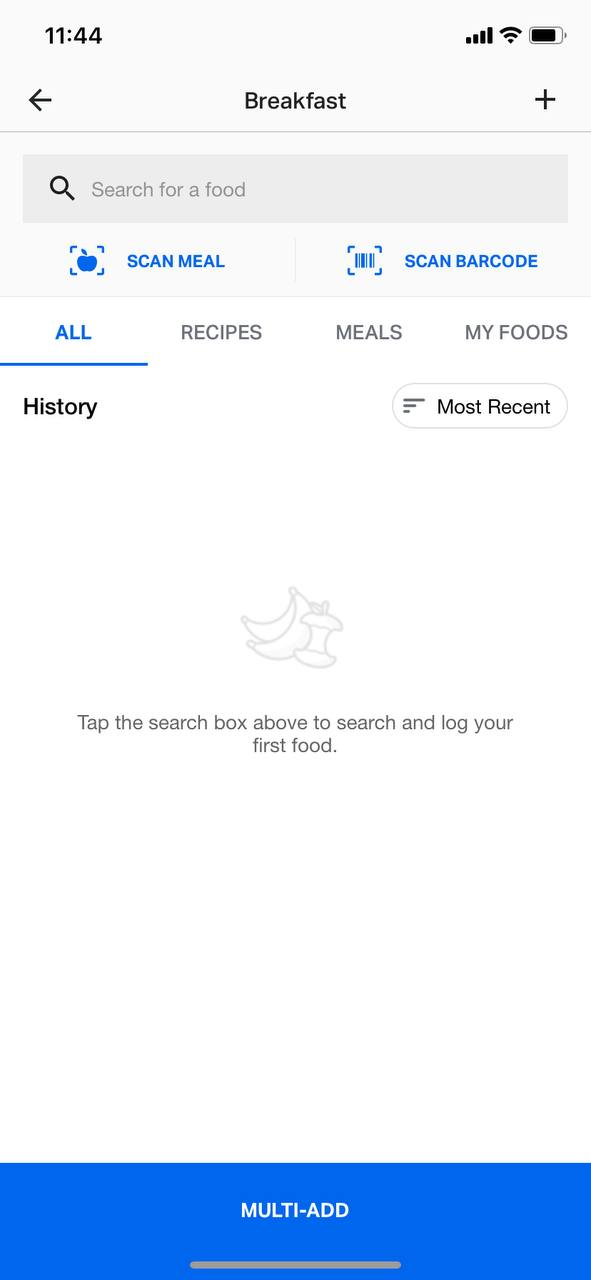A screenshot of a smartphone interface displaying a breakfast logging application at 11:44 AM. The top left corner shows the current time, while the right side of the screen displays indicators for cellular signal, Wi-Fi connectivity, and a nearly full battery. Immediately below, there is a navigation bar with a left arrow on the left, the word "Breakfast" centered, and a plus sign on the right.

Beneath the navigation bar is a gray line followed by a search bar with placeholder text reading "Search for a food" in gray. Below this search bar, there are two blue buttons labeled "Scan Meal" and "Scan Barcode."

Further down, there are three tabs labeled "All," "Recipes," "Meals," and "My Foods." The "All" tab is highlighted in blue, while the others are black. A blue line underlines the "All" tab. 

Below this section is a "History" heading, with a button labeled "My Most Recent" to the right. Underneath, there's an instructional text in gray advising, "Tap the search box above to search and log your first food."

The central part of the screen features a gray outline illustration of two bananas and an apple core. At the bottom, a blue stripe runs across the screen with the text "Multi-add" in white in the middle. Below this, a gray bar is present, which appears draggable.

The entire interface uses a color scheme primarily consisting of black, white, gray, and blue.